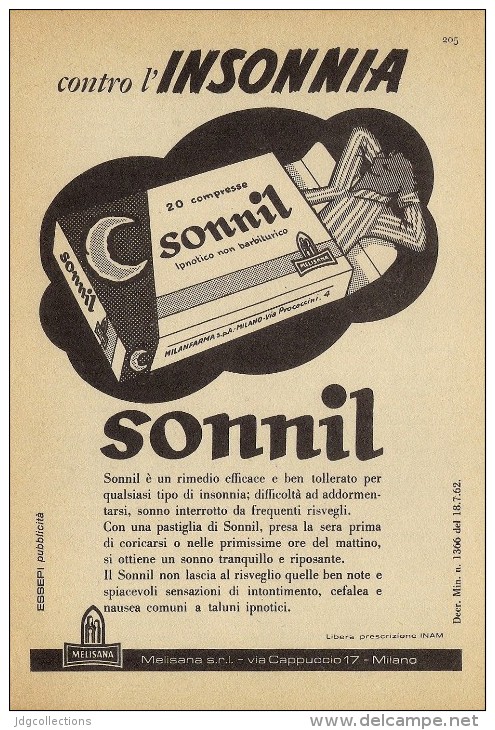The image depicts an old advertisement for a sleep aid product, probably from around 50 to 60 years ago, written in a foreign language, possibly French or Italian. The main text at the top reads "Contrôle de l'insomnia," indicating it is intended to manage insomnia. The color scheme is a dull, pale brownish-yellow with black text. Central to the ad is a cartoonish illustration of the upper half of a man dressed in striped pajamas, lying inside an open pill box labeled "Sunil." The box, which appears like a bed, features a half moon and the words "20 compress," suggesting it contains twenty pills. Below the illustration, the product name "Sunil" is prominently displayed, followed by a descriptive paragraph about the medication. In the lower left-hand corner, there is a logo likely representing the manufacturer. The overall style of the ad reflects typical vintage medicine advertisements.